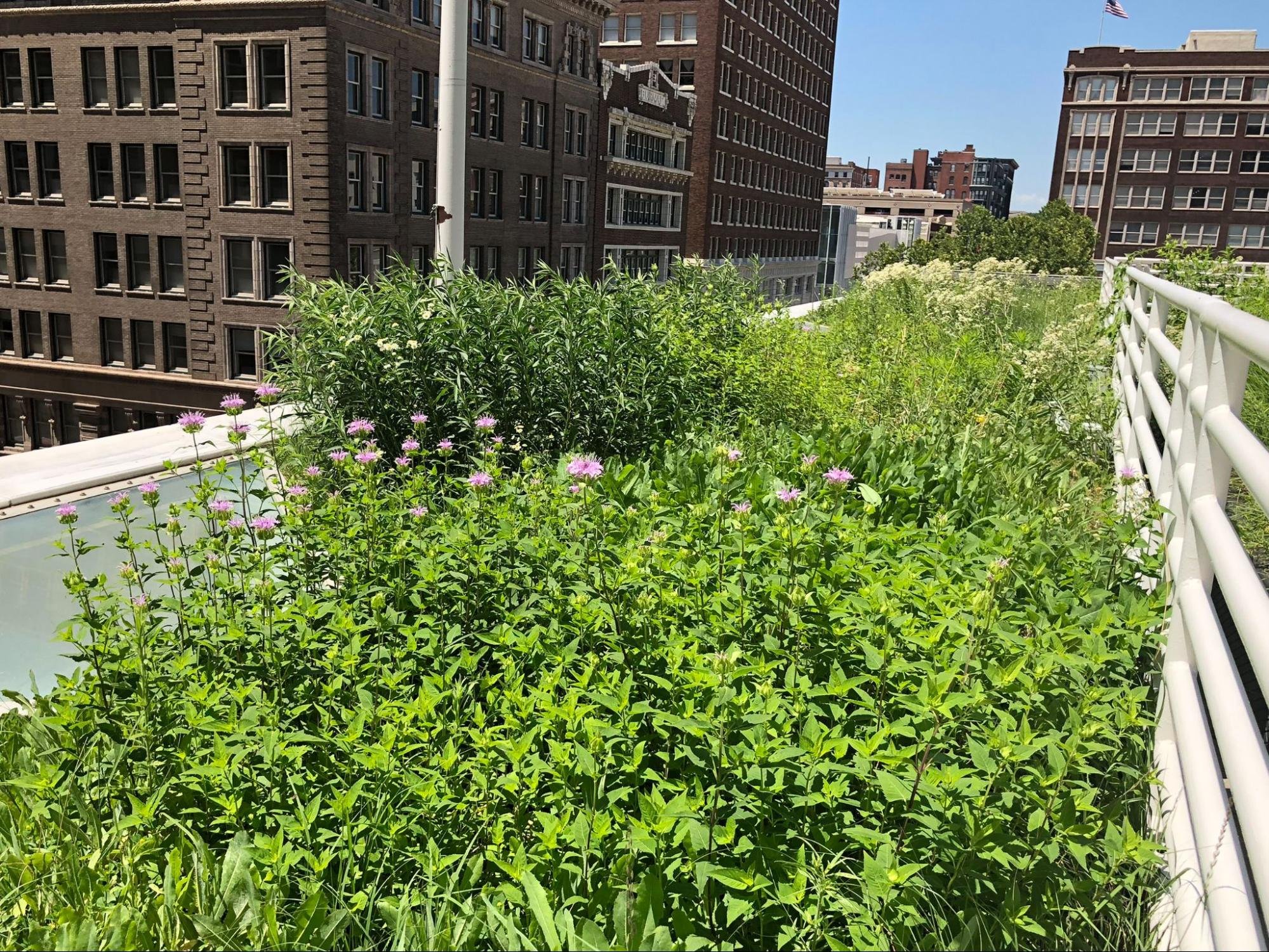The image depicts a sunny, cloudless day in an urban setting, possibly in a city like Chicago or New York City. We're looking at a rooftop garden situated on a building that isn't as tall as the surrounding structures. The neighboring buildings, which are primarily brown brick with numerous windows, extend several stories high and may serve as businesses or apartments. The garden itself is lush and somewhat overgrown, featuring an array of green plants with some pink and purple flowers. To the right of the garden is a white fence, approximately eight feet tall with eight links. Further in the background, a brown brick building can be seen flying a small American flag, subtly suggesting the garden's location within the United States.